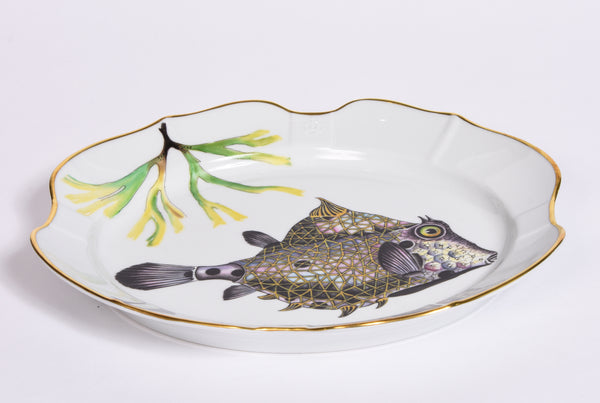A striking image showcases a white ceramic designer collector plate, distinguished by its gold-embossed, textured rim resembling an uneven ripple, almost shell-like in form. The plate, almost an inch deep, features a meticulously detailed depiction of a large brown fish at its center. This lifelike fish, with yellow variegated gills, scales, and a distinctive yellow eye, also has a black tail and two black dots on its back. Adding to the aquatic theme, a vibrant painting of a piece of seaweed or seagrass—green and yellow in hue—adorns the top left side of the plate, creating a balanced and artful composition.